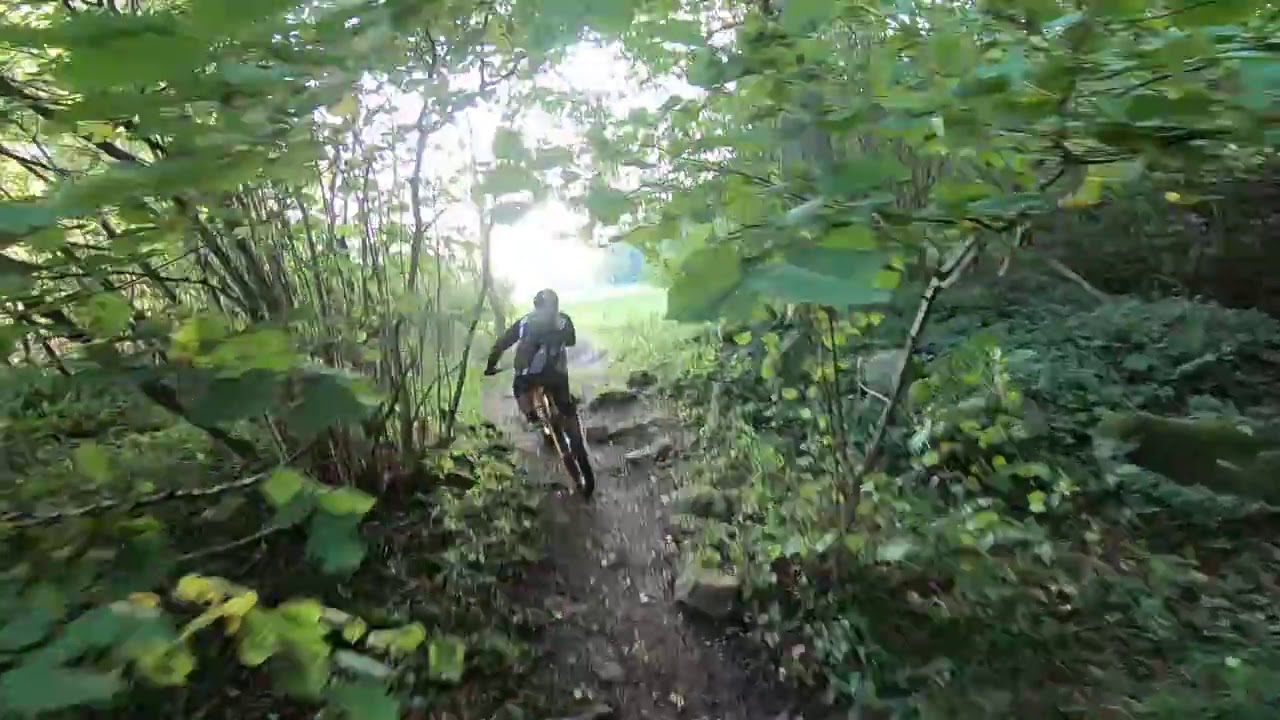This rectangular, horizontally aligned photograph captures a somewhat blurry scene of an individual bicycling away from the viewer through a dense, tree-lined nature trail. The dirt and rock path, narrow and slightly muddy, winds through abundant greenery with large rocks prominently lining the right side of the trail. The cyclist, seen from behind, is wearing a helmet and a dark gray or black long-sleeve top with either shorts or rolled-up sweatpants. Surrounding the trail are thick bushes, trees, and various weeds that partially enclose the path. In the distance, the trail appears to widen and open into a less densely forested area with more grass, leading to a brightly lit expanse, where the nearly blinding white sunlight obscures further details. The lower right corner and the center of the image are particularly blurry, adding to the dreamy, almost etheric quality of the scene.